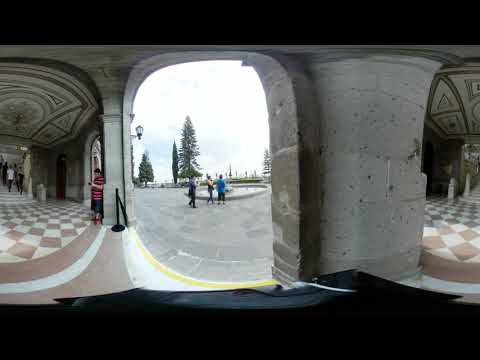The image captures a sophisticated and intricately designed structure from the perspective of someone inside, looking out through a curved archway entrance. On the left side, the ground features a white and brown checkered pattern and some sections with pink and white diamond shapes. The ceiling is meticulously adorned with various drawings and relief carvings, adding to the grandiosity of the scene. A man in a red and black striped shirt, black pants, and red shoes is seen leaning against the wall, seemingly focused on his cell phone.

In the middle of the image, the arched opening reveals an outdoor scene with a cloudy white sky and green trees in the background. A gray paved area, likely a square, is visible with a circular structure, possibly a fountain, around which three individuals are walking. The overall ambiance resembles an opulent underpass or pavilion, capturing both the grandeur of the interior and the serene simplicity of the exterior.